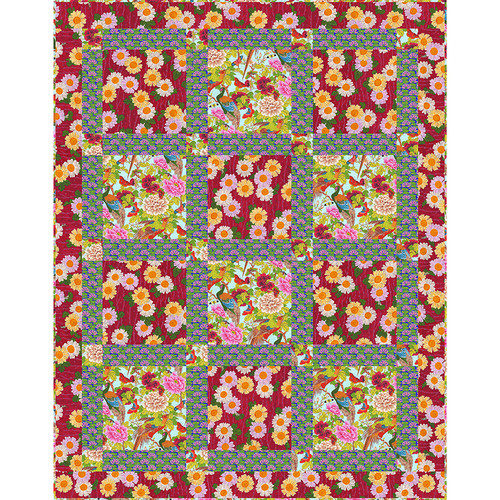This image features a large, rectangular quilt that dominates the entire frame. The quilt is primarily composed of a vivid red background adorned with a detailed floral pattern. The flowers on this red fabric include white, blue, pink daisies with orange centers, as well as orange, cream, and beige florals, all accompanied by green leaves. Interspersed within this main fabric are twelve distinct squares. Each of these squares is bordered in a combination of gray and pink hues. Six of these squares showcase an intricate design featuring birds and flowers. The birds, one with an orange breast and dark head and another that is red, are depicted sitting on brown stems with green leaves. Some of these squares also present flowers with a blue background, adding more variety to the design. Behind these floral squares, additional fabric behind features blue tones with pink and green florals, though this portion appears more subdued compared to the vibrant quilt front.